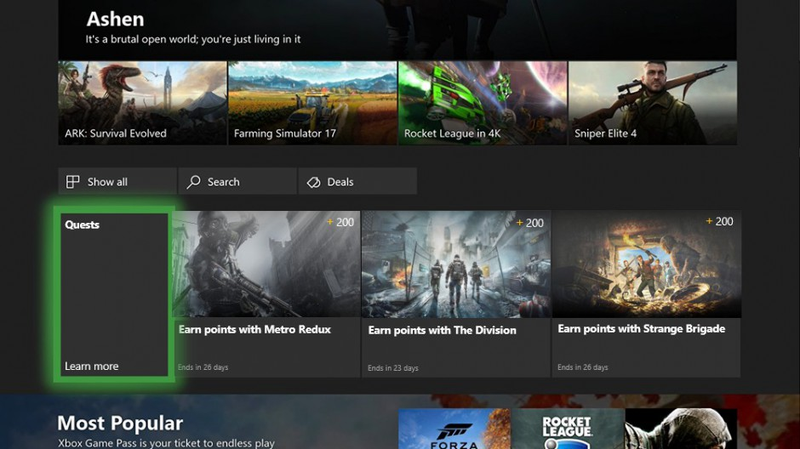The image showcases the Windows operating system's main menu bar, specifically opened to the gaming menu. Dominating the top portion is the word "Ashen" accompanied by a subheading that reads, "It's a brutal open world, you're just living in it." Below this header is a row displaying four game options with corresponding thumbnails: "Ark: Survival Evolved," "Farming Simulator 17," "Rocket League in 4K," and "Sniper Elite 4."

Further down, there are additional menu options labeled "Show All," "Search," and "Deals." Beneath these options is a rectangular section titled "Quests," with a prompt to "Learn More."

On the right-hand side of this section, there are three additional action items, each featuring a thumbnail and an option to earn 200 points: "Earn Points with Metro Redux," "Earn Points with The Division," and "Earn Points with Strange Brigade." Finally, at the bottom of the image, partially cut off, is an advertisement for popular games under the subheading "Xbox Game Pass," touting it as your ticket to endless play.